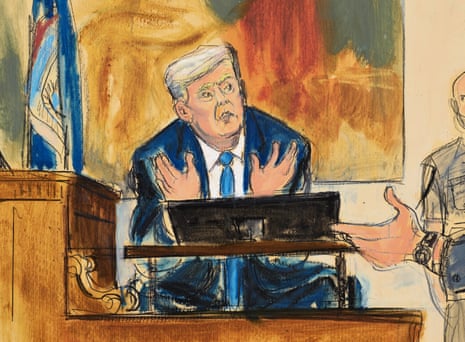In this detailed gouache courtroom drawing, Donald Trump is depicted on the witness stand with his hands raised near chest level. He is wearing a blue suit, white dress shirt, and a blue tie, his expression directed towards a gesticulating hand adorned with a watch, which likely belongs to a lawyer making a point. To Trump's right, a partial image of a security guard in blue is visible, his face partially obscured. Accompanying the scene is a flag featuring blue, red, and white elements, and a large, indistinct painting that forms the background. The drawing utilizes a palette of oranges, rusts, greens, blues, and pink flesh tones, highlighting the courtroom setting indoors. Trump is depicted in front of a black screen, possibly a tablet, reinforcing the technological context of the contemporary courtroom scenario.